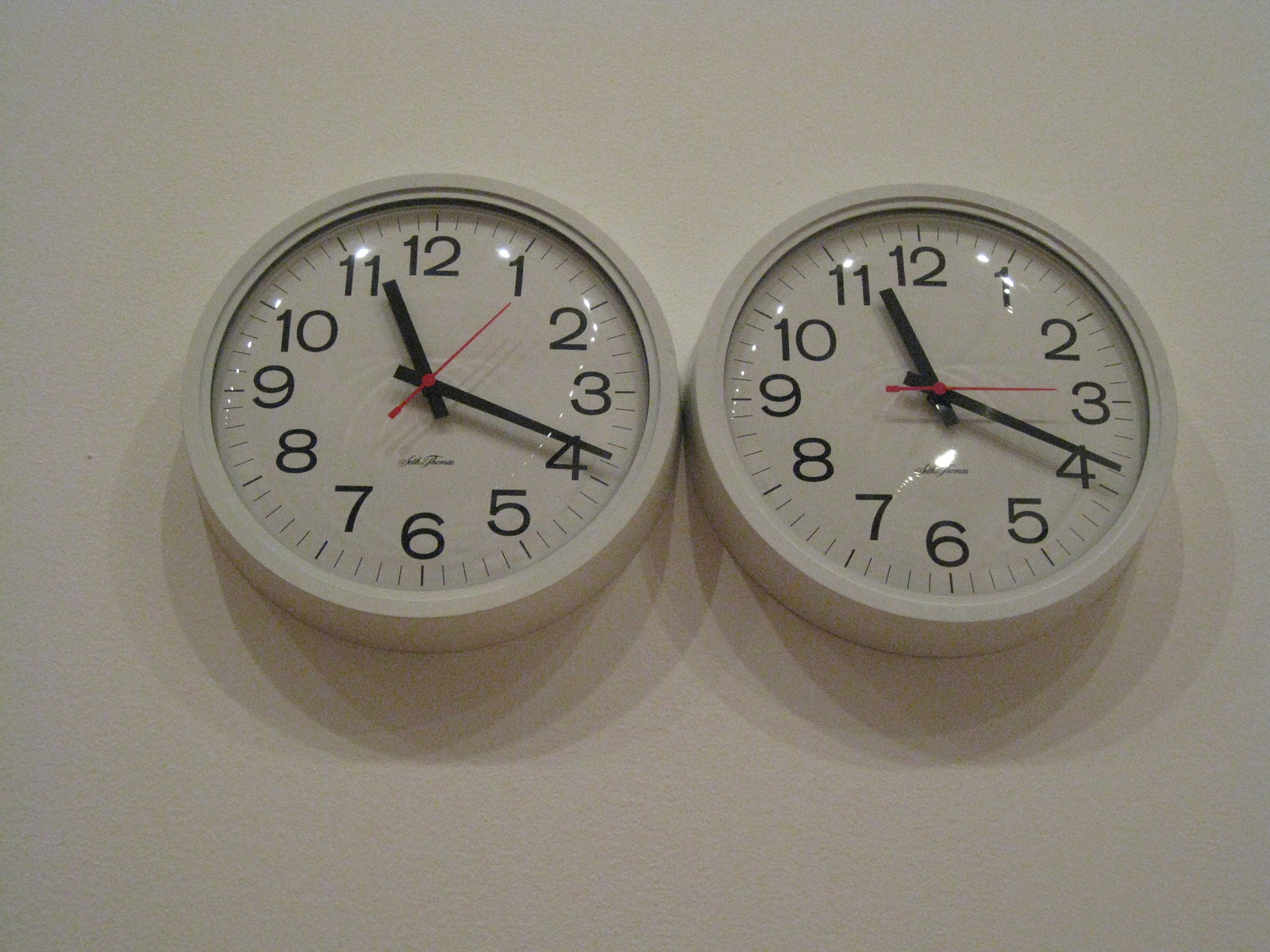This color photograph depicts two identical clocks mounted side-by-side on a plain white wall. Both clocks feature a white casing and white faces, covered with glass. The black numerals and clock hands stand in stark contrast against the white background, with the exception of the red second hand on each clock. The clock on the left displays the time as approximately 11:18, with its red second hand positioned at the 1. The clock on the right also shows approximately 11:18, but its red second hand is at the 3. Gentle shadows are cast beneath each clock, adding a subtle depth to the otherwise minimalist scene. The image is devoid of any text.